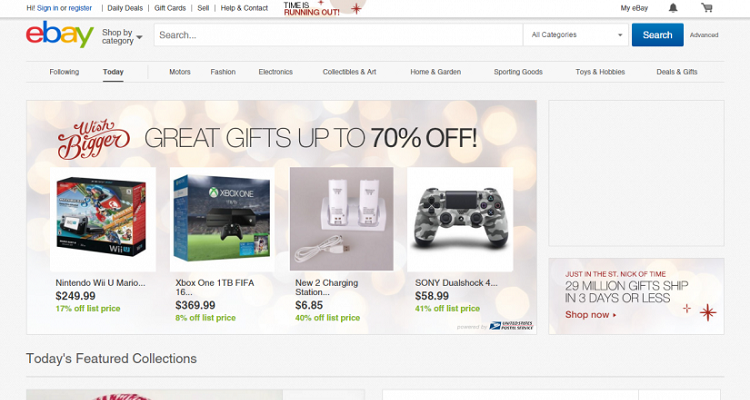**Detailed Caption:**

The image depicts a computer screen displaying the eBay homepage. At the very top of the screen, the options "Hi! Sign in or register" are visible. Adjacent to these options are various site navigational links including "Daily Deals," "Gift Cards," "Sell," "Help & Contact." 

There is a promotional banner situated prominently at the top with the message, “Time is running out” followed by a stylized plus sign. Moving towards the right of the top bar, you can see "My eBay," a black notification bell icon, and a shopping cart icon.

Beneath this top section, the main eBay logo is present, featuring a red 'e', a blue 'b', a yellow 'a', and a green 'y'. The central portion of the page provides a "Shop by category" dropdown menu, a search bar with the placeholder text "Search...", and a dropdown to toggle between different categories. A blue rectangle button labeled "Search" is at the end of the search bar, with an "Advanced" search option further to the right.

The lower portion of the screen showcases the "wish bigger great gifts up to 70% off" promotion. Featured items include images of a Nintendo Wii U Mario game, an Xbox One FIFA game, new charging stations, and a Sony DualShock controller.

This detailed layout illustrates both navigational elements and promotional content designed to attract and guide users through the shopping experience on eBay.